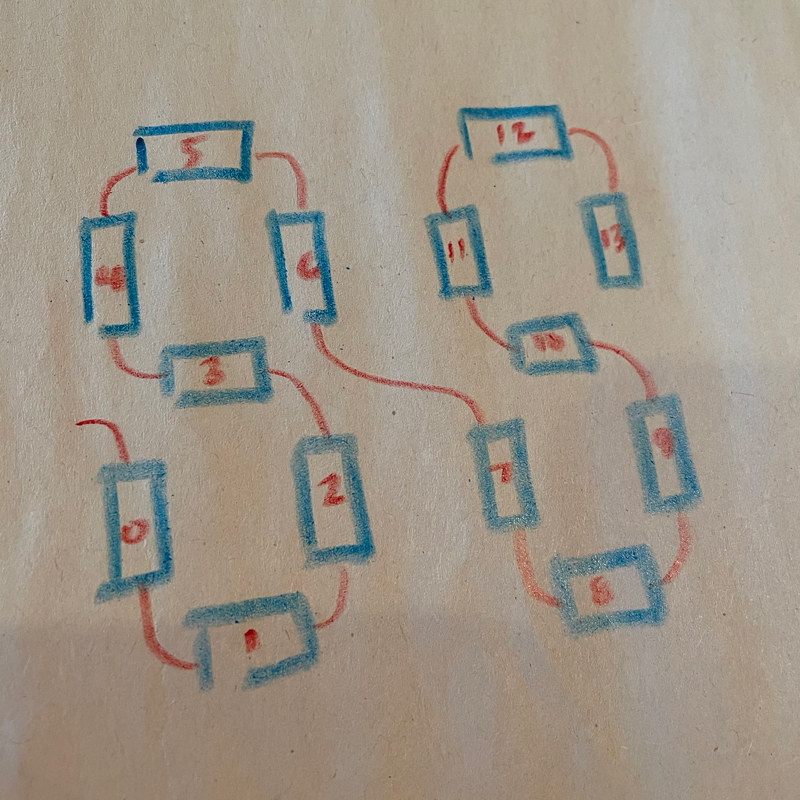The photograph captures a hand-drawn piece of art created with either markers or crayons, rendered on a beige piece of paper reminiscent of the inexpensive brownish paper often used in schools. The drawing consists of intertwining squiggly red lines and blue rectangles, alongside red numbers that guide the viewer through the intricate design. The squiggly lines resemble the shapes of two connected S's. Beginning at the bottom tail of the first S, there is a blue rectangle labeled '0'. Following the line counterclockwise leads to another rectangle marked '1' near the bottom curve of the S. 

As you continue upwards, the next blue rectangle encountered is labeled '2'. Ascending further around the middle part of the S, '3' is positioned. On the upper left side of the S is '4', while the apex of this first S is designated as '5'. Descending again, '6' is next, before crossing over to the second connected S at the lower right where '7' is found. The base of this second S contains '8', and moving upwards along the right curve, '9'. In the middle of the second S is '10', with '11' located on the left side. Finally, the top of the second S is marked '12' and descending to the final rectangle brings you to '13'. The use of vivid colors and playful lines creates a captivating and whimsical visual journey across the paper.